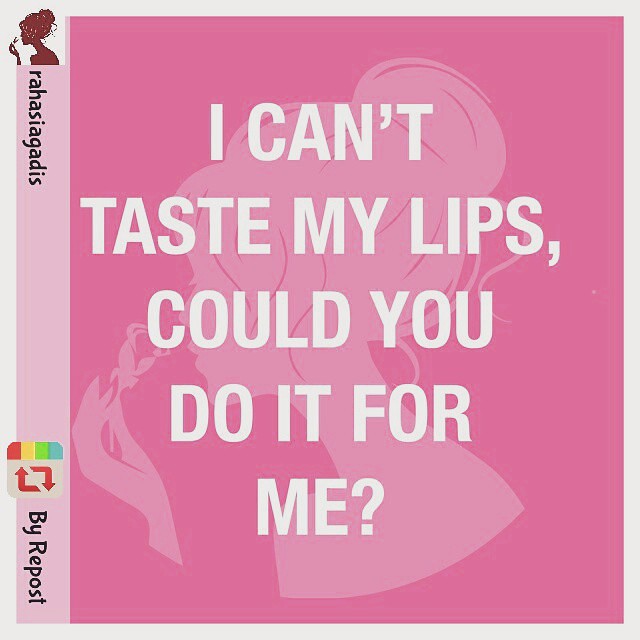The image is a square visual often found on social media or Pinterest, featuring a two-tone pink background with white text. The background is predominantly a medium pink, adorned with a lighter pink silhouette of a woman with her long hair pulled up, sideways, and appearing to smell a rose. The central quote reads in white text, "I can't taste my lips, could you do it for me?" On the very left of the image is a vertical light pink strip, which separates the main visual from additional elements. At the top of this strip, there is a handle, "Rahasiagoddess," accompanied by a small logo of the woman smelling the rose. Towards the bottom of the strip, there is a colorful repost icon with the words "by repost" written in black. The overall design is framed with a white border, enhancing the visual appeal.